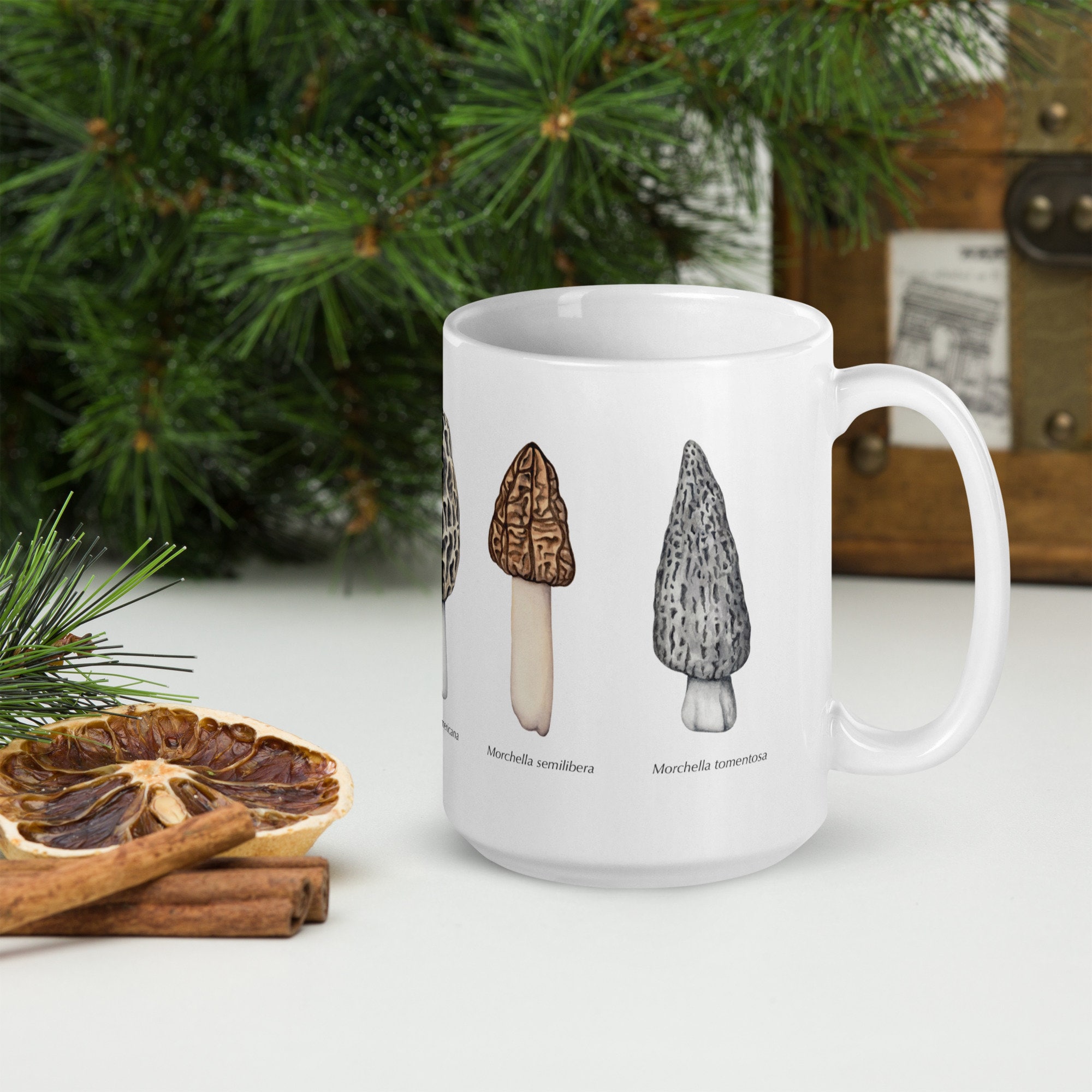This photograph captures a serene and festive scene centered around a white ceramic mug adorned with detailed illustrations of various mushroom species. The mug, slightly taller than a standard one, prominently displays two fully visible mushroom sketches: a brown, textured Morchella semilibera with an off-white stem, and a grayscale Morchella tementosa with a shorter stem. Each mushroom is labeled just underneath its respective image.

The mug sits on a pristine white tabletop. To its left, an artistic arrangement includes a slice of dried citrus fruit, likely a blood orange, alongside a cluster of cinnamon sticks and a scattering of pine needles, contributing to a warm, rustic aesthetic.

In the blurred background on the left side of the image stands a lush, green pine tree reminiscent of Christmas, while on the right side there appears to be an antique wooden trunk adorned with metal buckles and studs, adding a touch of vintage charm to the composition. The overall focus remains on the elegantly adorned mug, but the surrounding elements enhance the cozy, festive atmosphere of the scene.